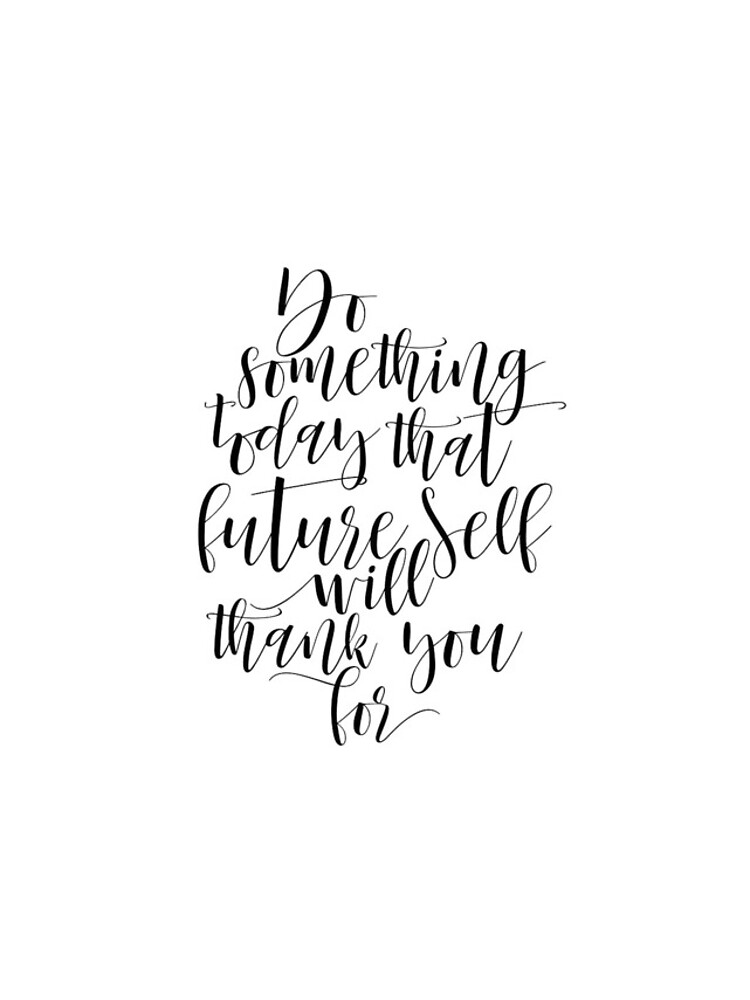The image features a motivational quote presented as black script on a white background. The text, formatted in a decorative and flowy cursive font, appears center-aligned and reads, "Do something today that future self will thank you for." Each word is positioned on a separate line, collectively forming a vertically elongated oval-like shape. The script gives an impression of being somewhat disorganized, with varying letter heights and exaggerated loops and flourishes, lending it a handwritten, organic feel. Despite the elaborate font and uneven baseline, the text remains readable and visually centered.